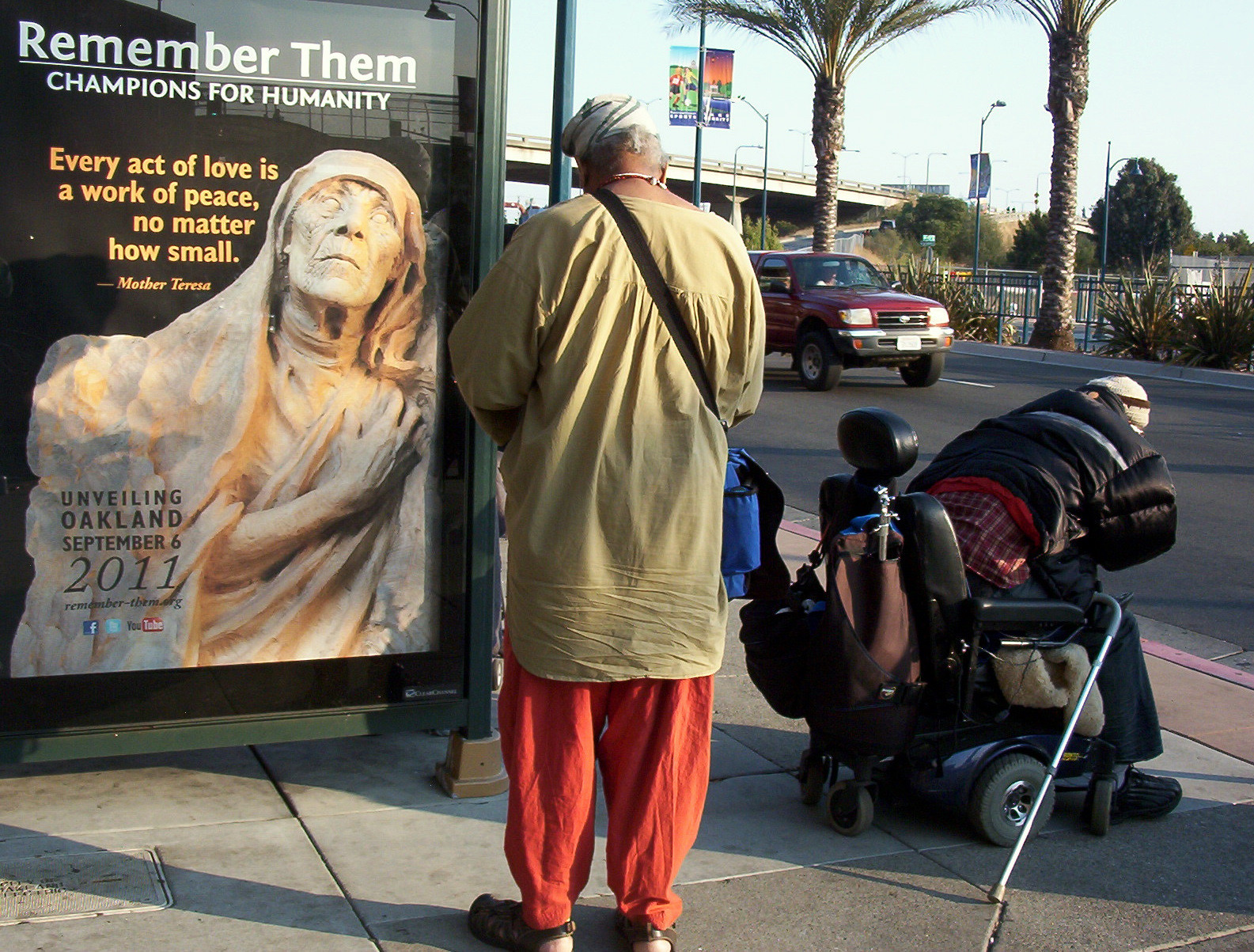This detailed street scene captures a vibrant and diverse moment at a bus stop in Oakland, California. Dominating the left side, there's an advertisement on the bus shelter Plexiglas for a Mother Teresa exhibit titled "Remember Them: Champions for Humanity" with her quote, "Every act of love is a work of peace, no matter how small." It commemorates the unveiling in Oakland on September 6, 2011. The poster features a statue of Mother Teresa clutching her chest, enveloped in a scarf. 

In the foreground, on the right side, a man with brown skin and distinct ethnic attire stands. He dons a light green, long, flowy top coupled with red or pink baggy pants, and a scarf wrapped around his head, suggesting a Persian or another cultural influence. He also carries a blue shoulder bag. Adjacent to him is another man, seated in an automated wheelchair adorned with black leather padding and a cane beside him. He is hunched over, wearing a large black coat, seemingly waiting for the bus. 

The backdrop features a clear blue sky and an overpass bridge. Palm trees line the center of the busy street, giving a tropical feel reminiscent of southern cities, Hawaii, or Florida. Adding to the lively urban atmosphere, a colorful purple truck can be seen driving by.